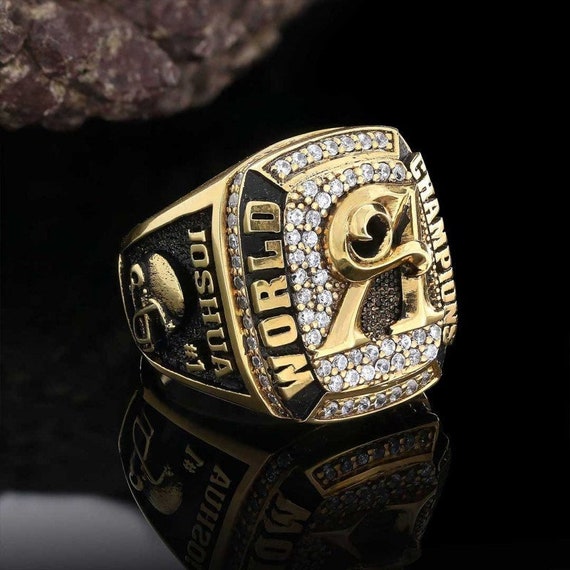The image features a large, gold, championship-style ring, typically associated with sports victories. The ring, clearly designed for a man, prominently displays a bold, swirly "A" encrusted with numerous small clear stones, likely diamonds, which also form rows on the top and bottom of the "A." Surrounding the letters on the face, the ring announces "world champions" in engraved text. The ring's band is etched with the name "Joshua" and the phrase "number one," accompanied by the image of a football helmet. The ring has a chunky, square shape and is photographed resting on a high-polished, black, shimmery surface, which reflects the ring's form and the ambient light, enhancing its glass-like shine.